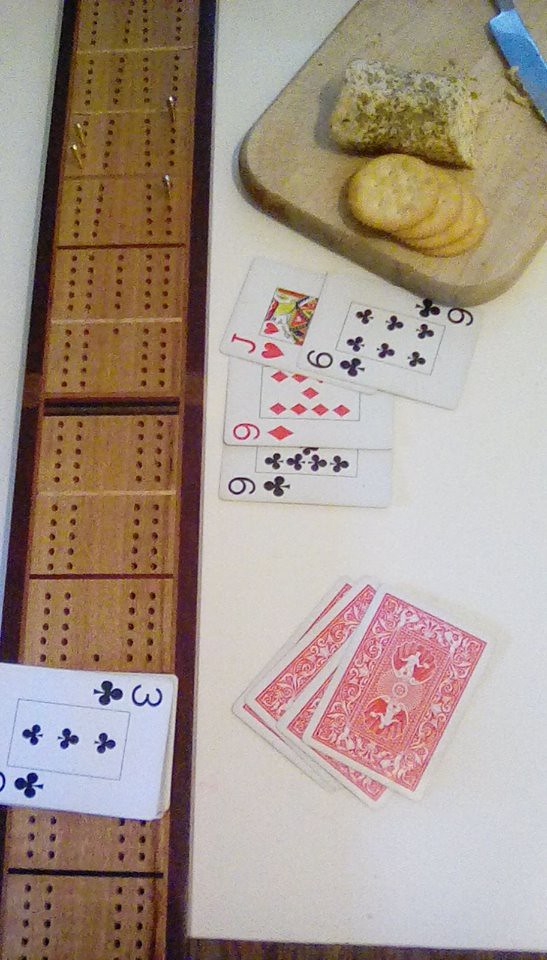This photograph captures a white table meticulously arranged with various items. On the left side of the table sits a wooden P-knuckle counting board, adorned at the top with four gold pins. The board itself is perforated with numerous holes and divided into sections marked by yellow and red lines, transitioning into segments of whole wooden pieces. 

At the bottom left corner lies a card showing the three of clubs, resting atop a small stack of additional cards. To its right, a separate set of three or four cards is placed face down, their red backs featuring a white design of a person raising their hand. 

Above these, a sequence of playing cards—nine of clubs, nine of diamonds, jack of hearts, and six of clubs—are displayed in a neat row. Directly above this row sits a charcuterie board adorned with three or four round crackers and a cheese ball, complemented by a silver knife positioned at the top right corner of the board.

The white tablecloth covers most of the table but is slightly disrupted at the bottom edge of the photograph, revealing a strip of the underlying wooden surface.